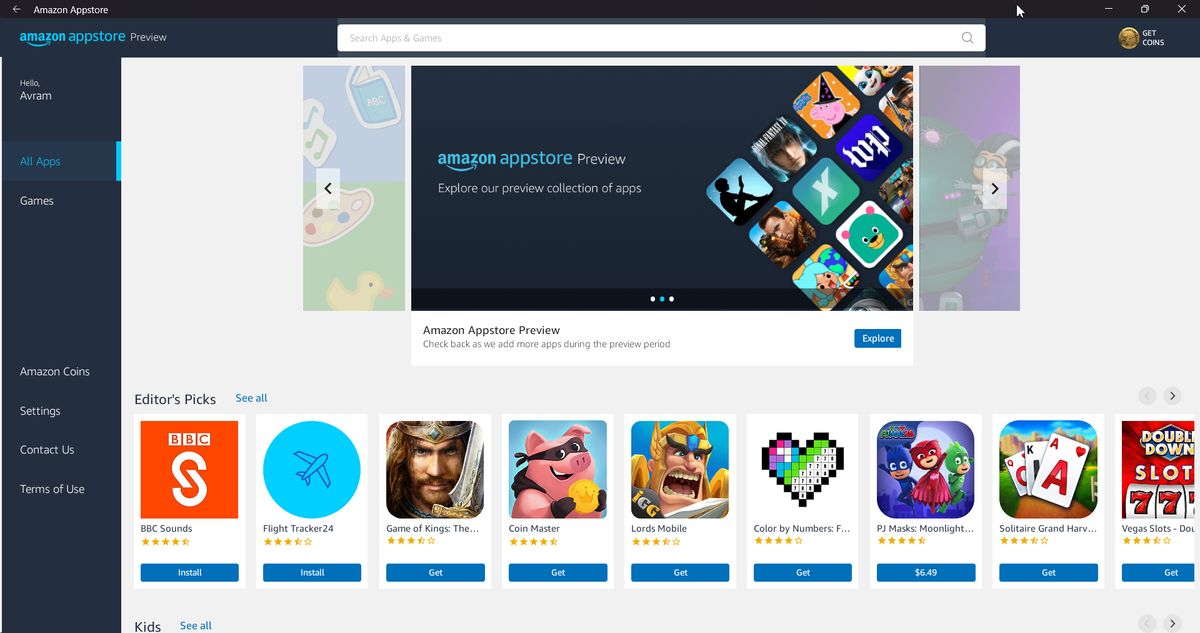Screenshot of the Amazon App Store Preview:

In the upper left-hand corner, white text on a black border prominently displays "Amazon App Store." The top right-hand corner features the standard Minimize, Maximize, and Close (X) icons. 

Below this header, a navy blue border contains the text "Amazon App Store Preview," with a white search bar and a Get Coins icon on the right-hand side. 

On the left-hand side of the screen, there is a vertical navy blue sidebar with white text, stating "Hello AFRAM" (spelled out as A-V-R-A-M). The sidebar also includes menu options: All Apps, Games, Amazon Coins, Settings, Contact Us, and Terms of Use.

The central part of the screen displays another "Amazon App Store Preview" area. This section invites users to explore the current collection of apps in a carousel-style window showcasing various app icons. A text prompt underneath advises users to "check back as we add more apps during the preview period." A prominent "Explore" button encourages further browsing.

Below this, there is an "Editor's Pick" section with a "See All" link for more recommendations. Featured apps in this section include:
- BBC Sounds
- Flight Tracker 24
- Game of Kings
- Coin Master
- Lords Mobile
- Color by Numbers
- PJ Masks Moonlight
- Solitaire Grand Harvest
- Vegas Slots

This well-organized layout offers users a preview of the app selection and encourages them to explore more features and offerings.